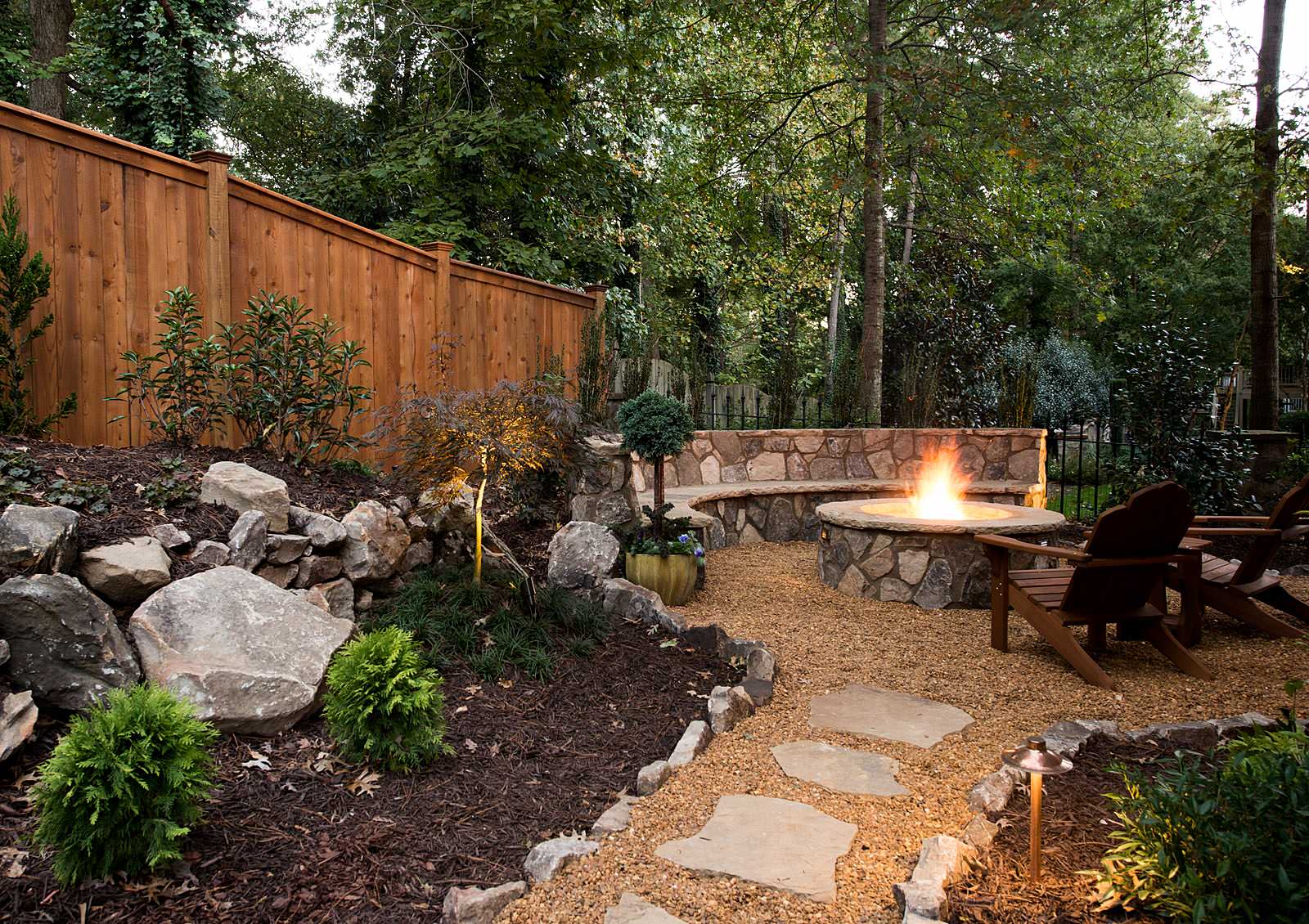This image portrays a serene backyard setting, likely belonging to a high-class residence. Dominated by a prominent wooden fence in a rich brown mahogany color in the top left corner, the scene leads down a sandy path interspersed with silver and gray square cobblestone steps. At the heart of the backyard, there is a cylindrical stone fire pit with a vibrant active fire emitting hues of orange and red. Surrounding the fire pit are two dark brown, stained wooden chairs with armrests, designed for relaxing while facing the fire. Additional seating includes a stone bench. The area is bordered by short rocky walls housing small plant gardens, adding to the picturesque and tranquil environment. The backdrop features tall, dark gray trees with bright green leaves, suggesting a forest or wooded area beyond the backyard’s confines.